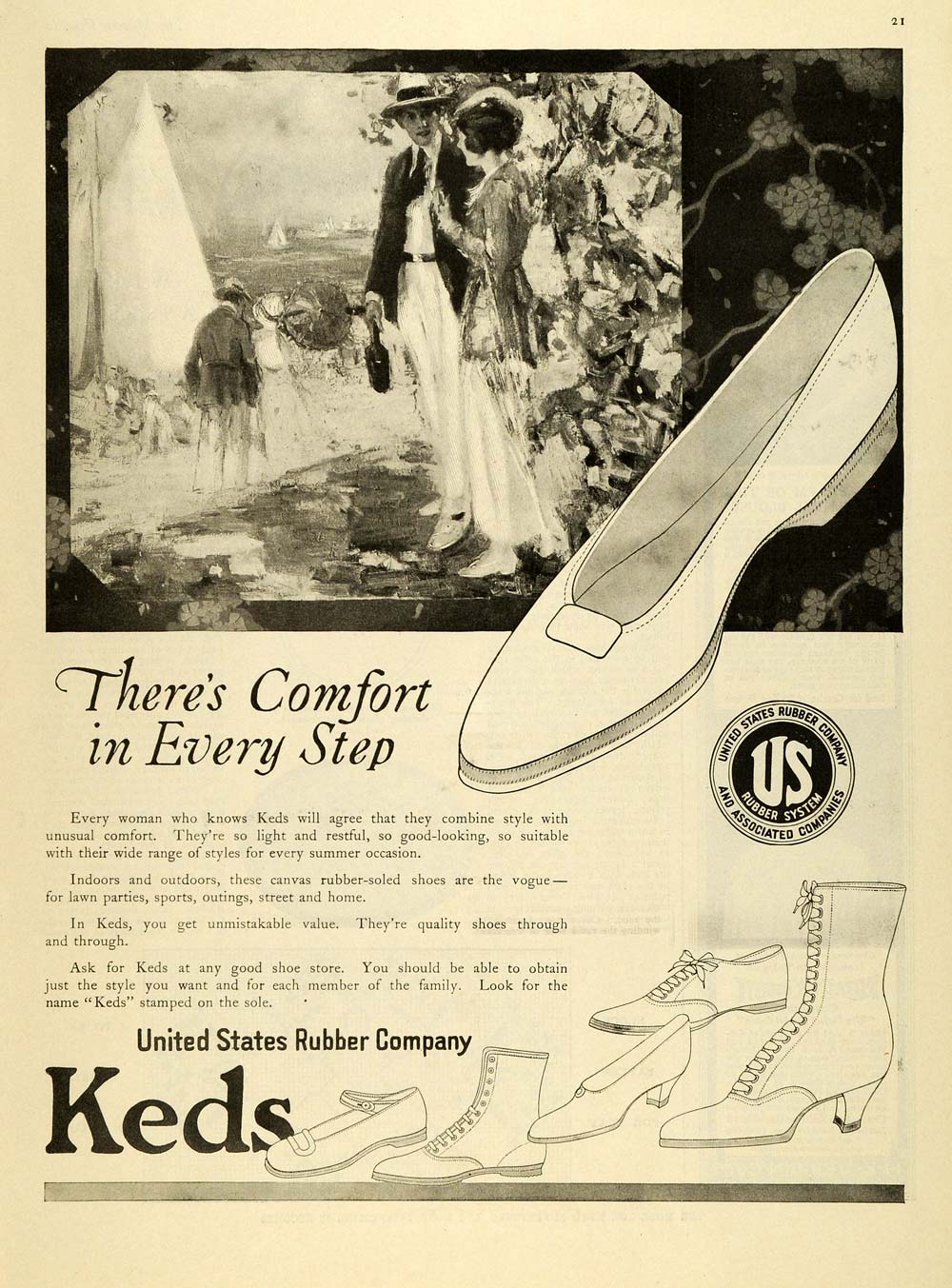This detailed black and white full-page advertisement, appearing on page 21 of an old, yellowed magazine, promotes Keds shoes by the United States Rubber Company. The ad is dominated by an elegant black and white oil painting at the top, depicting a stylish couple in period clothing from the early 20th century. The man, wearing a white fedora with a black ribbon, a black suit jacket, white pants, a white shirt, and white shoes, stands beside a woman with short flapper-era hair, dressed in a sweater over a dress and carrying an umbrella. In the background, people are seen strolling towards a beach dotted with sailboats.

Beneath this image, a large illustration of a low-heeled, slip-on woman’s shoe is featured prominently on the lower right. Overlapping this advertisement is the statement in bold text, "There's comfort in every step." The detailed text extols the virtues of Keds shoes, highlighting their combination of style and comfort, their lightweight, restful nature, and their suitability for varied occasions such as lawn parties, sports outings, and everyday use. The ad assures consumers of the quality and value of these canvas rubber-soled shoes and suggests they look for the Keds name stamped on the sole.

An appeal to "Ask for Keds at any good shoe store" emphasizes that the shoes are available in a wide range of styles for every family member. Finishing the ad, several smaller black and white illustrations of different shoe styles are displayed, including Mary Jane shoes, dress shoes, boots, and Oxford shoes. The advertisement also features the logo and text, "United States Rubber Company, Keds," along with mention of the "U.S. Rubber System and Associated Companies."